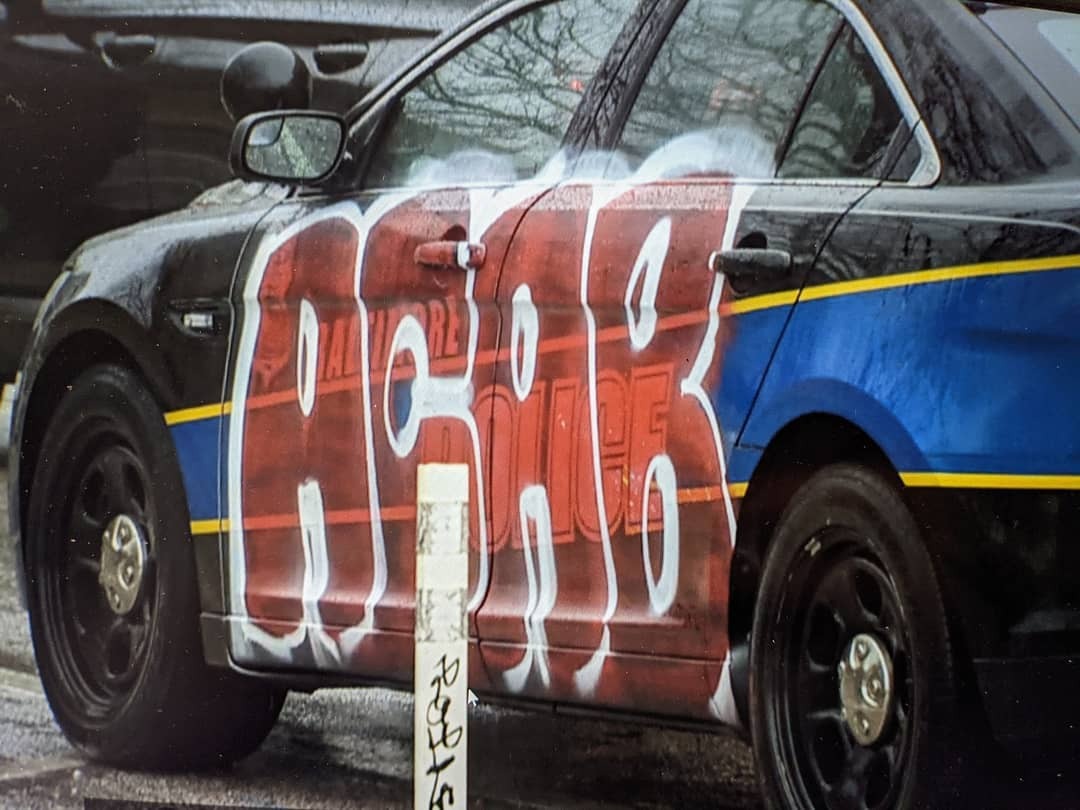A detailed description of the image would be:

A black police sedan marked with the text "BALTIMORE POLICE" in all capital letters on the side. The lettering is accompanied by a blue streak outlined in yellow that extends from the front wheel well to the trunk of the vehicle. Vandalism has occurred, as someone has spray-painted the acronym "ACAB," which stands for "All Cops Are Bastards," over the police markings. The graffiti is done in red paint with a white outline, written in a rounded, bubble-style font with the letters slightly squished together and entirely in uppercase. Despite the defacement, the original "BALTIMORE POLICE" logo remains visible underneath the spray paint.